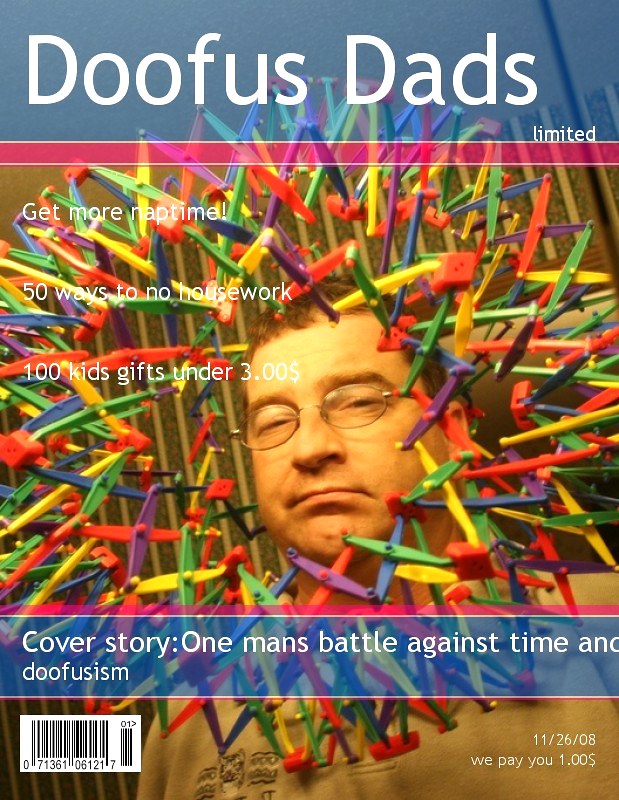This is a detailed description of a magazine cover titled "Doofus Dads Limited" with a barcode in the lower left corner and the date November 26, 2008, in the lower right corner alongside the text "We pay you one dollar." The cover features a photograph of a man with short brown hair, thick brown eyebrows, and small-rimmed glasses. The man has a smirk on his face and is adorned with an elaborate, colorful construction of interconnected sticks in blue, green, red, purple, and yellow, draped around his head and neck. The title "Doofus Dads" is prominently displayed in white lettering on a bluish background at the top of the cover. Additional text on the cover includes tips like "Get more nap time," "50 ways to no housework," and "100 kids' gifts under $3," in white lettering that's somewhat difficult to read. Beneath the man's face, on a light bluish background, is the cover story title: "One man's battle against time and doofism."